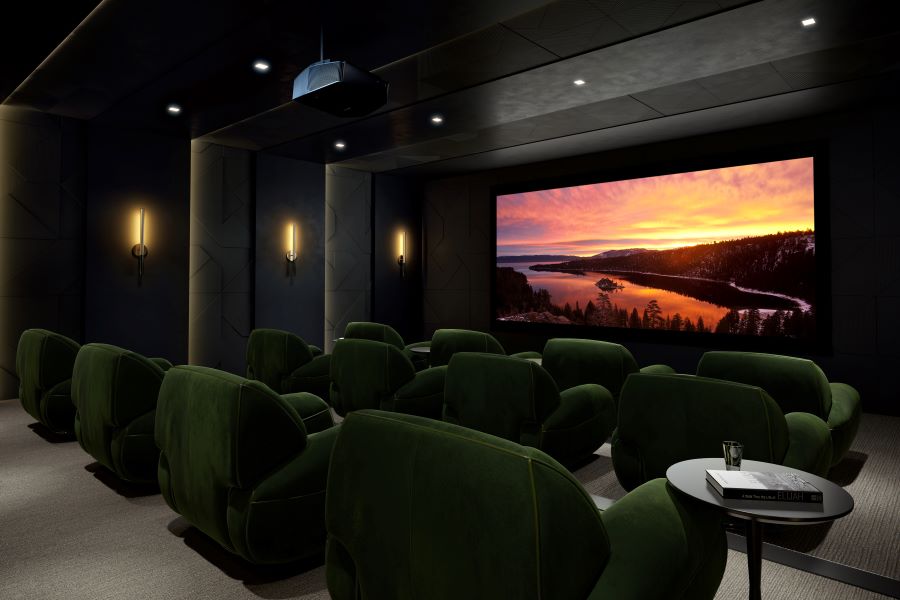This image captures the ambiance of a luxurious home theater adorned with twelve oversized, exceedingly comfortable chairs arranged in two rows, each with a green tint. The dark atmosphere of the room is accentuated by theater lighting along the sides, casting a soft glow against the walls and ceiling, both painted black to enhance the cinematic feel. The gray carpeted floor adds to the overall elegance of the space. Dominating the front of the room is an enormous screen built seamlessly into the wall, currently displaying a mesmerizing scene featuring a river meandering through a landscape of small shrubs and grass, with mountains silhouetted against a radiant sunset sky. Hues of orange, yellow, blue, and reflective metallic grays pervade the scene, creating a vivid and immersive viewing experience. On the right-hand side of the room sits a small black circular table, holding a book and a disposable coffee cup, adding a touch of lived-in comfort to the luxurious setting. This high-end, inviting theater room combines sophistication with coziness, making it an ideal spot for enjoying movies.